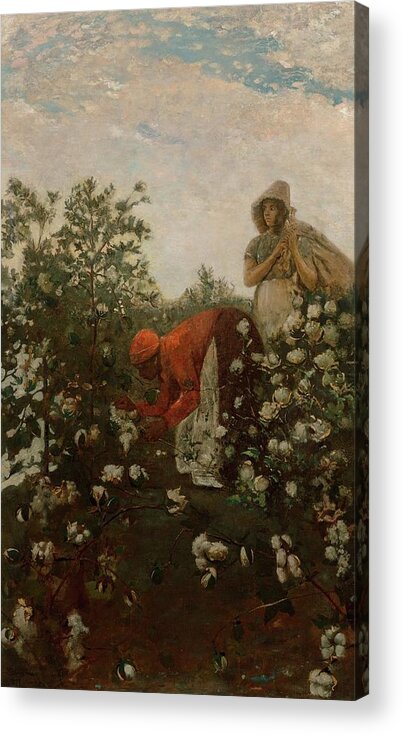This detailed vintage-style painting captures a daytime scene of two women picking cotton in a field under a sky filled with clouds interspersed with streaks of blue. The foreground features an African American woman, bent over, diligently picking cotton. She is adorned in an orange blouse with a brown ankle-length skirt and a white apron. Her head is wrapped in an orange bun-style cap that keeps her hair neatly in place.

Standing directly behind her is a woman of European descent. She is wearing a straw hat that extends down to her shoulders, providing shade as she works. Her attire consists of a pale blue dress, a white apron tied around her waist, and she carries a sack over her left shoulder. The woman gazes off to the right, likely overseeing their progress in the cotton field filled with an abundance of the fluffy white crop.

The painting, rendered on a fabric board style frame, imbues a sense of timelessness, capturing the essence of labor and the human condition in an era gone by.